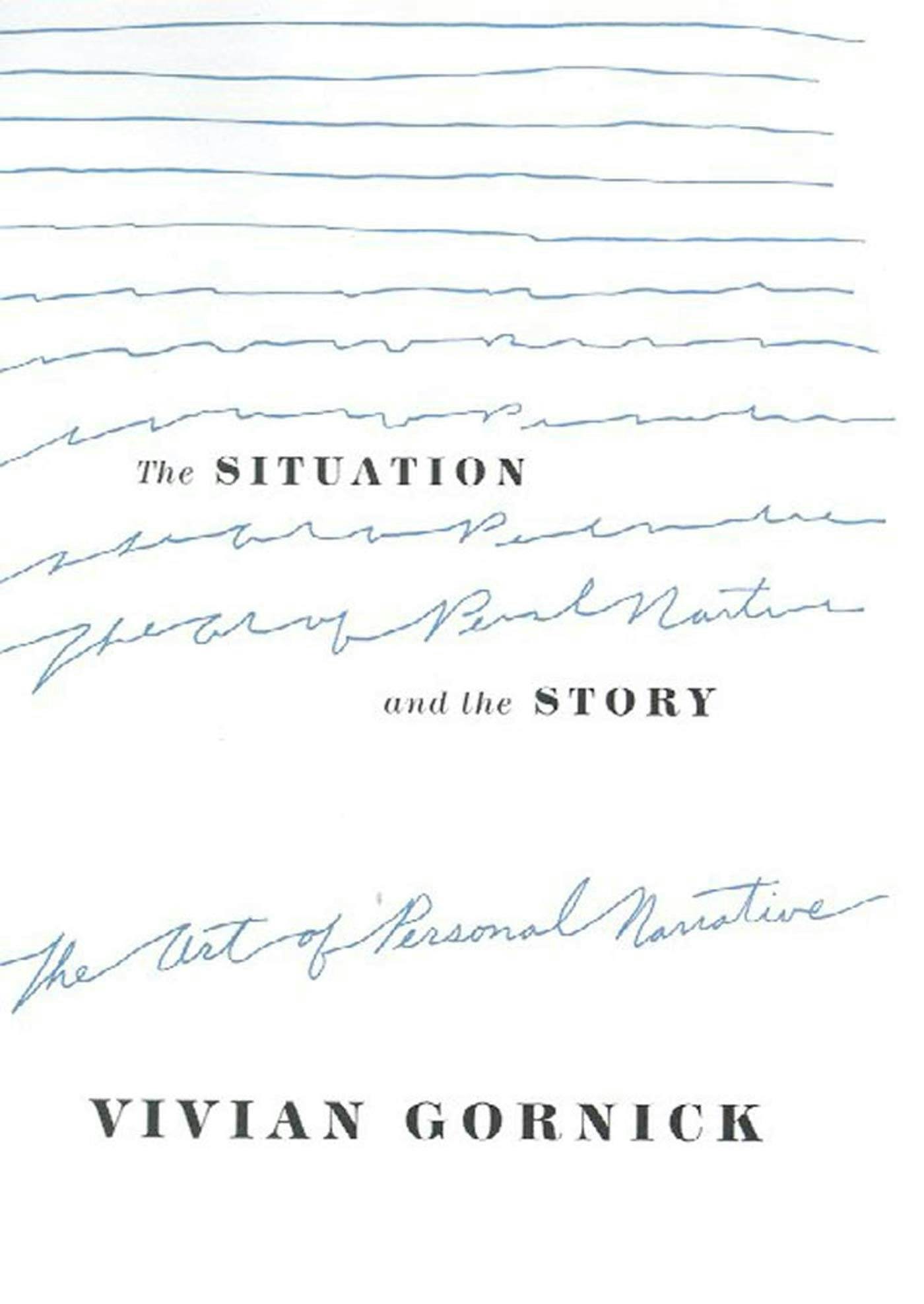The image appears to be the white cover of a book, featuring predominantly black and dark blue writing. At the top, bold black text reads "The Situation," followed by a few squiggly lines that evolve into cursive writing as they descend. This cursive transforms from mere squiggles to almost legible text, among which the phrase "the art of personal narrative" becomes clearer towards the bottom. In between, more bold black text states "and the Story." The name "Vivian Gornick" is prominently displayed in bold at the bottom. The overall design gives an impression of lines transitioning from straight and orderly to more fluid, as if written freehand on notebook paper.